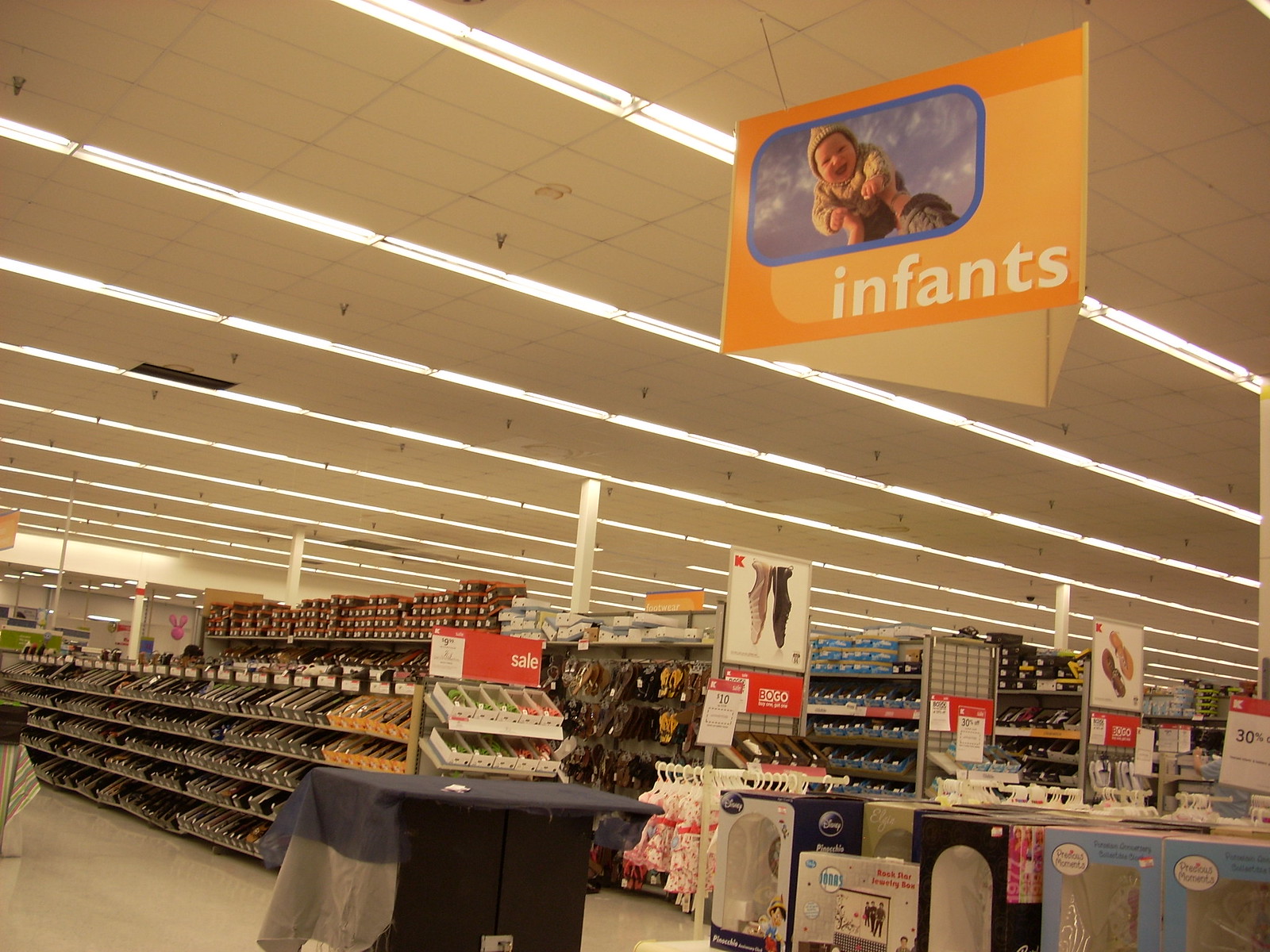This detailed color photograph captures the interior of a large department store, specifically within the shoe and infants' clothing sections. The image is taken from eye level, angled slightly to the side, allowing a partial view down several aisles. The aisle closest to the camera features shelves filled with variously colored shoe boxes, predominantly yellow and orange. The adjacent aisle has items hanging, likely socks, and a sign above indicating shoes.

Further down, another aisle contains numerous shoe boxes, including black ones with blue boxes on the top shelf. The exact contents of the following aisle are unclear. In the foreground, there's a table draped in a blue and gray cloth. Suspended from the white ceiling, which is well-lit by long rectangular fluorescent lights, is a prominent orange and square-shaped sign designed to be visible from three angles. This sign depicts an infant being held up against a backdrop of a blue sky with clouds, and it features the word "infants" in white lettering, signaling the section's focus.

The store's vastness is emphasized by the numerous rows of shelves and racks extending into the distance, and the main aisle also displays stacks of items and clothing, including what appears to be children's garments on white hangers. The scene encapsulates the expansive and organized layout typical of a major clothing department store.